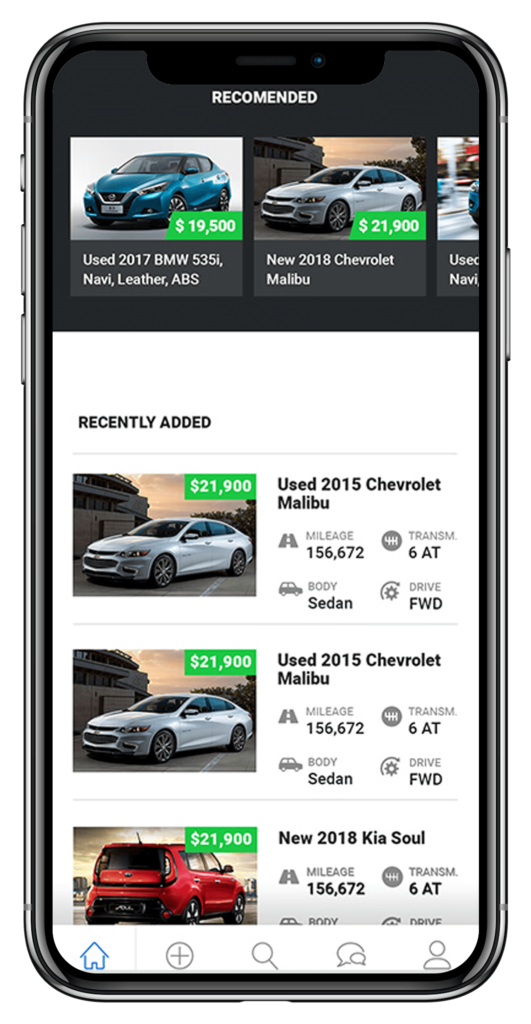The image features a cell phone encased in a light black, or dark grey, protective cover. On the left-hand side of this cell phone, there are three buttons: two larger volume buttons for raising and lowering the volume, and a smaller button located above them. On the right-hand side, there is a single, larger button.

The phone's screen displays a car purchasing website. At the top portion of the screen, occupying about 25% of the display, is a gray box labeled "Recommended." Below this, there are three boxes, each showcasing a car for sale, though the third one on the right is partially cut off from view. The first car listed on the left is a used 2017 BMW with a price tag of $19,500. To its right, the second car listed is a new 2018 Chevrolet Malibu, priced at $21,900. Beneath these listings, there is a white section entitled "Recently Added."